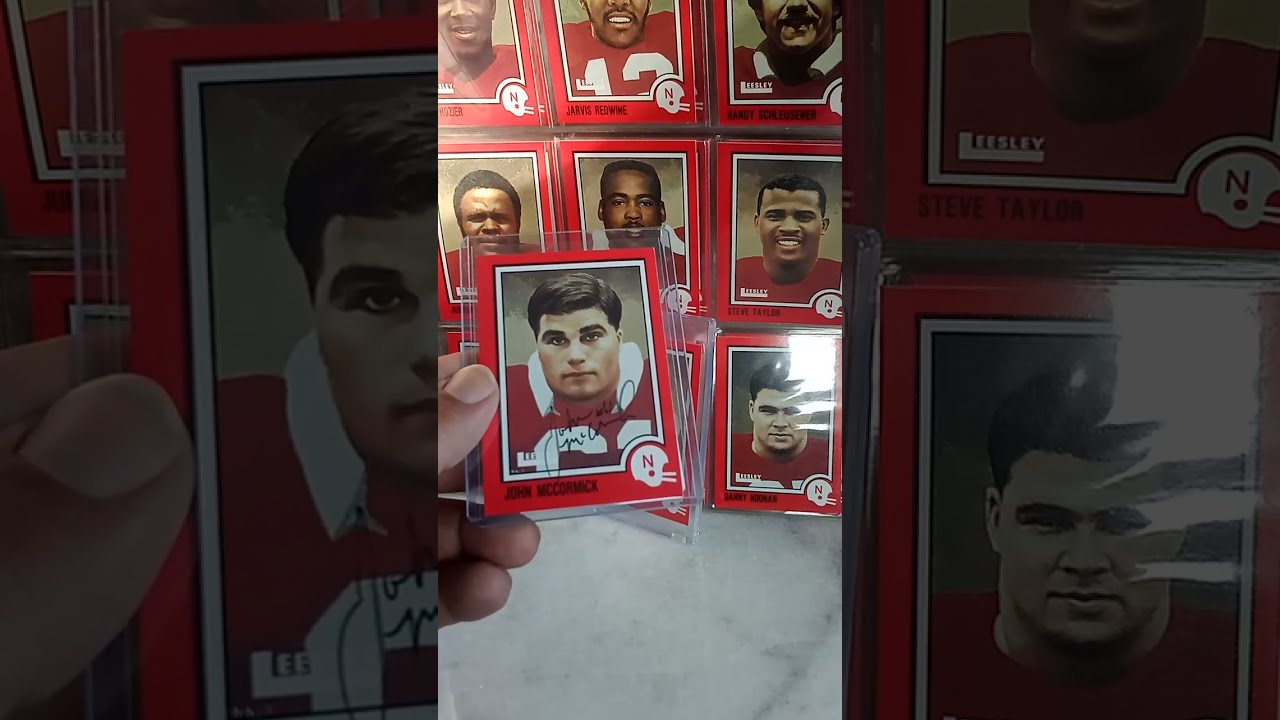The image features a color photograph, captured vertically on a cell phone, showing a collection of NFL football cards. The central focus is on a human hand, likely male, holding a specific card of a football player named John McCormick. This card, prominently displayed in the center portrait orientation, features a red border and a white inner border, with an image of the player donning a red jersey with a white collar. The card includes McCormick's signature across the front, along with a stylized football helmet logo bearing a red letter 'N' in the bottom right corner and the player's name in the bottom left.

Framing this central image are darkened black bars on either side, which overlay and enlarge the overall visual of the collection. Surrounding the highlighted card are eight additional cards, all depicting male football players in jerseys, a mix of black and white, and giving a vintage vibe reminiscent of the late 70s or early 80s. The arrangement showcases the diversity of the collection while emphasizing the details and nostalgia through the central image’s sharp focus and vivid colors.